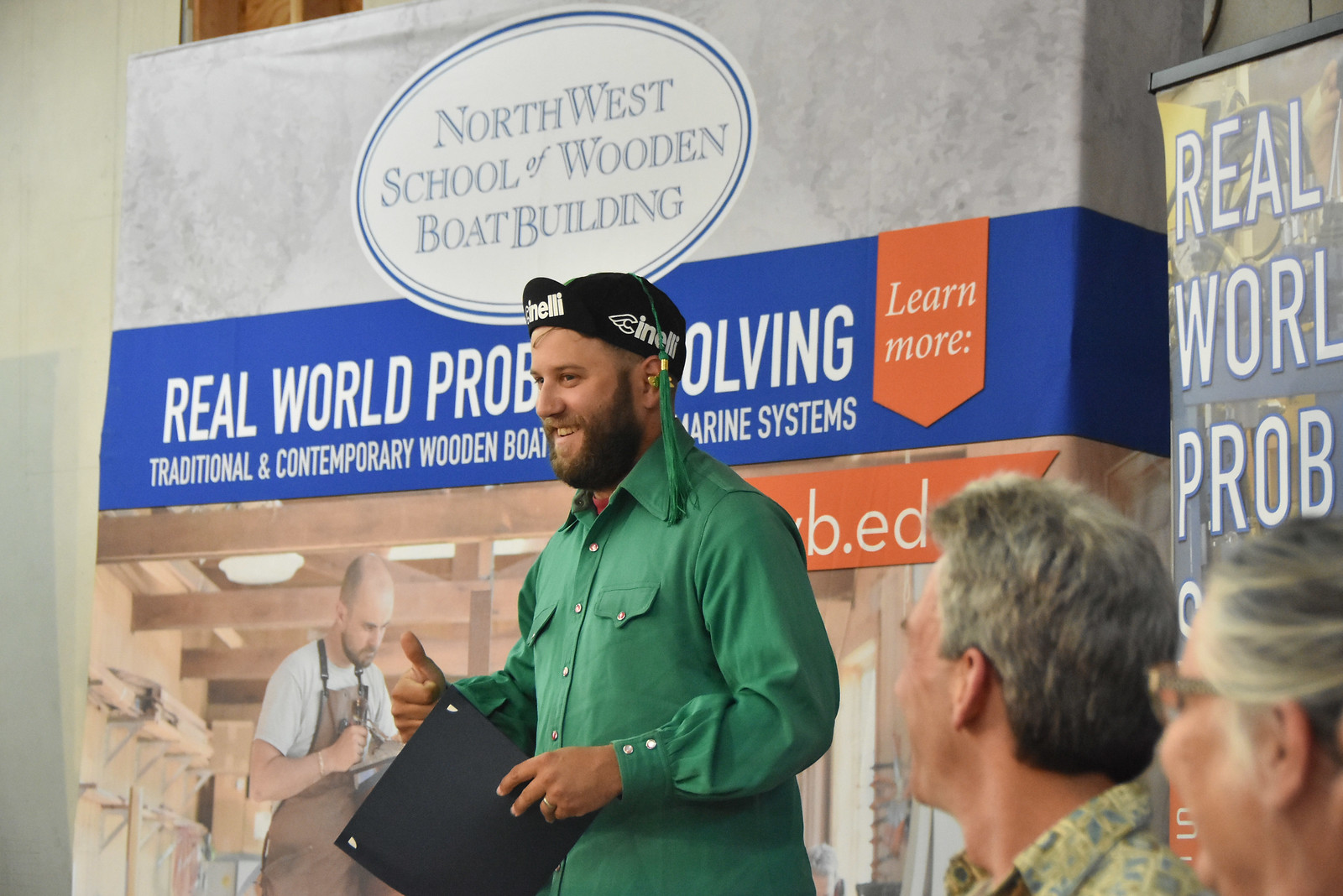In this image, we see a lively moment at a Northwest School of Wooden Boat Building event. In the center of the picture stands a light-skinned man, prominently featured from the waist up. He is preparing to present or receive a certificate, which he holds in his right hand, with hints of the document's white edges peeking out from the black folder. The man sports a green button-up shirt and a distinctive black Cinelli hat, with the cap flipped up and a green tassel hanging from it, suggesting it might be a graduation ceremony. His face beams with a smile, and a neatly kept beard frames his expression. Flanking him at the bottom right are two older people—a gray-haired man and a gray-haired woman in glasses—both looking up at him with pride and joy, possibly his parents. The background is dominated by a large promotional sign reading "Northwest School of Wooden Boat Building," adorned with additional text and a poster illustrating a man in an apron working in a wood shop.